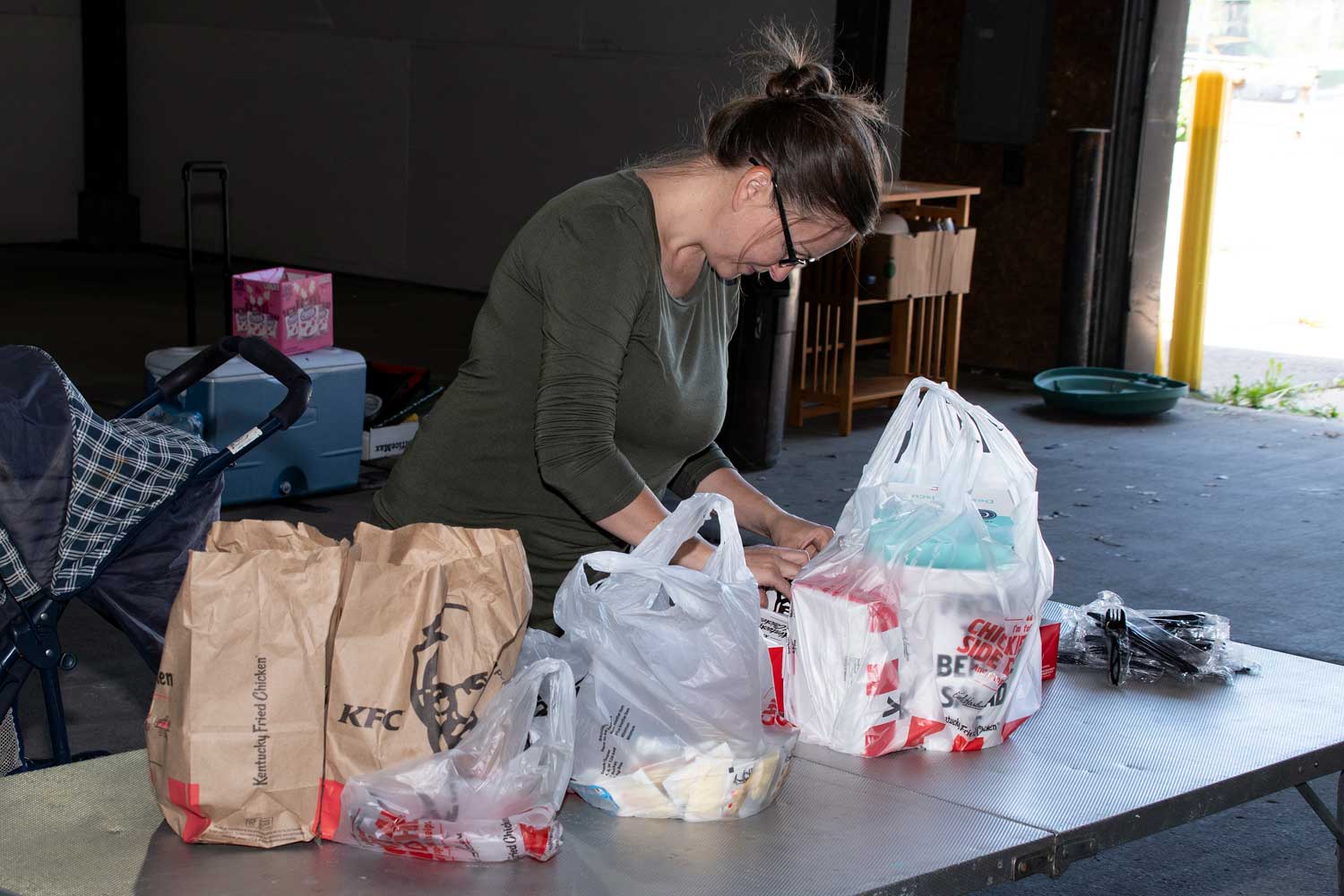In this detailed image, a woman with brownish hair wearing a green top and black-rimmed glasses is focused on a KFC pickup order in front of her. On the right side of the table, there are black forks and knives, and a clear plastic bag containing Kentucky Fried Chicken with its distinctive white and red color scheme. To her left, there are two more clear plastic bags; one contains brown paper bags featuring the KFC logo and text "KFC" in black, alongside another bag that reads "Kentucky Fried Chicken" with a hint of red at the bottom. 

Behind the woman, slightly to the left, is a baby carriage with a black handle, a blue base, and a checkered fabric pattern in green and gray. Also behind her is a blue and white-topped cooler, atop which sits a purple box. A yellow pole is visible on the right, next to a green bin lying on the ground. The flooring is gray, and the table resembles a silver folding table typically used in various indoor settings. A brown shelving unit is partially visible behind her, set against a grayish wall where the yellow pole is positioned.